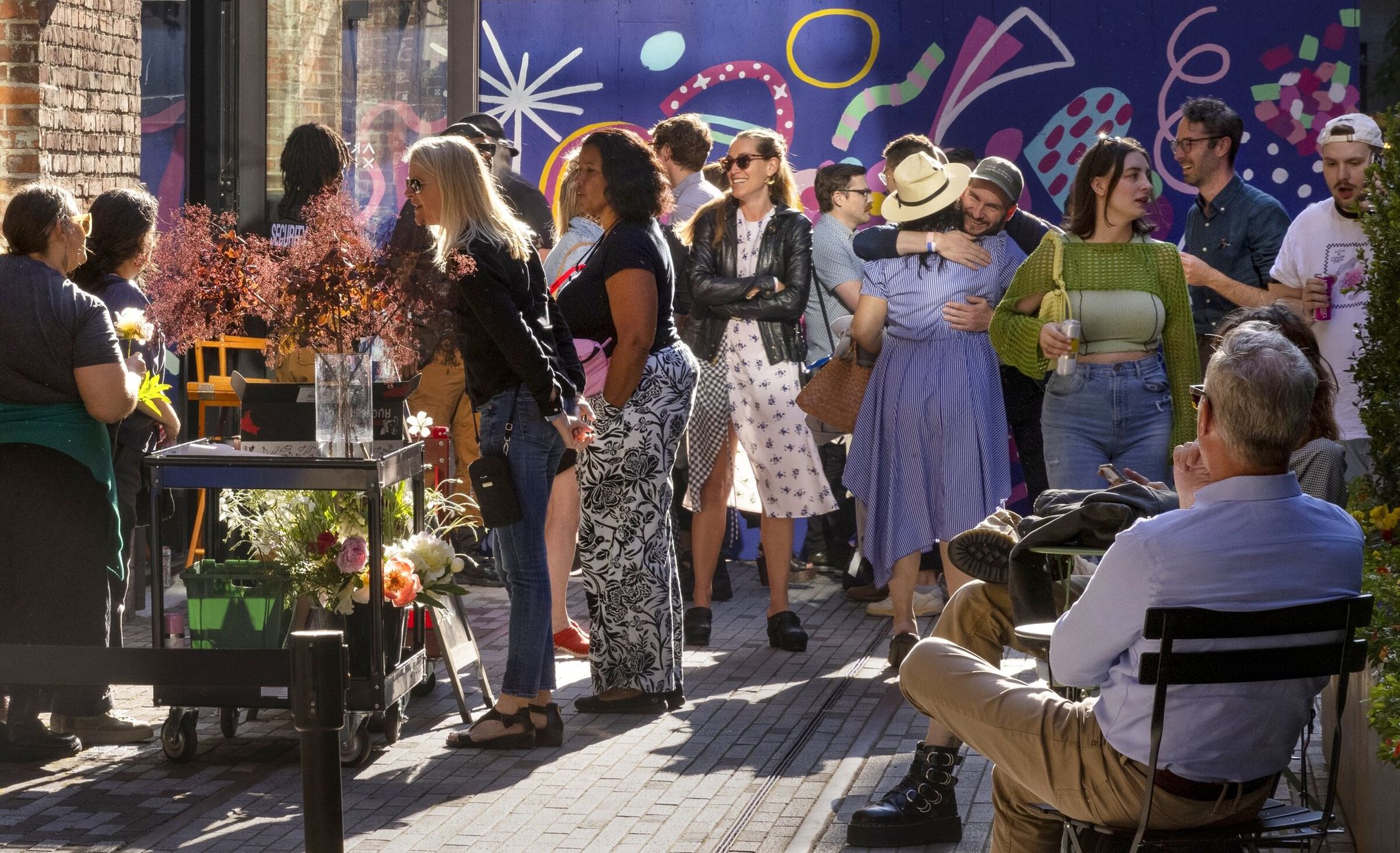The image captures a lively and joyful party setting, likely taking place in an outdoor courtyard or a cafe. The space is intimate, bustling with over a dozen people, some of whom are seated while others stand and mingle. The mood is cheerful, with most individuals greeting each other, hugging, and dancing. Many hold drinks, predominantly canned, adding to the festive atmosphere. 

In the foreground on the bottom right, a man sits with his back to the camera on a wooden chair, and near him, a woman whose features are not distinctly visible. The background reveals a mix of people, predominantly standing, chatting, and enjoying the gathering. To the left, two women are seen examining a mobile cart adorned with a glass vase containing red wildflowers, additional bouquets below in plastic containers, and individual flowers being held by other women, suggesting that flowers might be part of the celebration.

The setting is enhanced by the decor: brick walls on the left and a vividly colored, decorated wall in the background, plus wooden tables and chairs scattered around, some adorned with beautiful green and slightly reddish plants. The attire of the attendees is casually stylish, featuring a variety of light blue, green, black, brown, pink, orange, and gray colors, blending harmoniously with the daytime light that streams into the space. Overall, the photograph vividly conveys a scene of casual elegance and communal enjoyment.